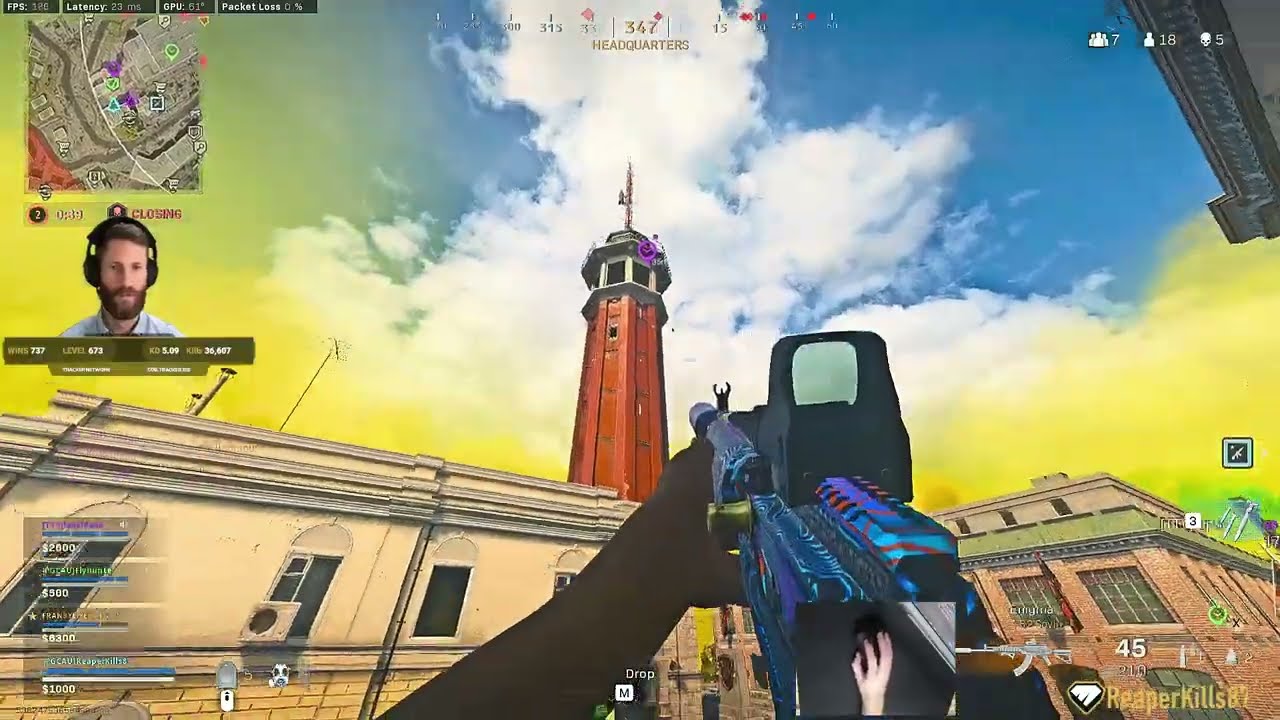This detailed screenshot from a first-person shooter video game captures a player's perspective looking up at a red octagonal tower with a white top and spire. The tower rises from a gray, rectangular building that spans the width of the image, and a brick building with multiple square windows is visible on the lower right side. The sky above is light blue, filled with puffy, wispy white clouds, some tinged with yellow and streaks of green. In the foreground, a pair of hands grips a colorful machine gun with a blue casing, red streaks, and a scope, aimed at the tower. 

Video game HUD elements populate the screen: the top-left corner features a mini-map with roads and various colored icons. Below it, a photo of a white man with a brown beard and short brown hair wearing headphones is displayed; this is likely the player. His stats, including 737 wins and level 673, are partially visible next to his image. Additional icons appear in the top-right and top-center areas of the screen. The bottom-left corner shows meters indicating amounts of money, while the bottom-right corner includes an icon of the weapon, some numbers, and possibly the phrase "Reaper kills." Just right of the center bottom area, a smaller photograph shows the player's hand on a black mouse, emphasizing the live gameplay aspect.